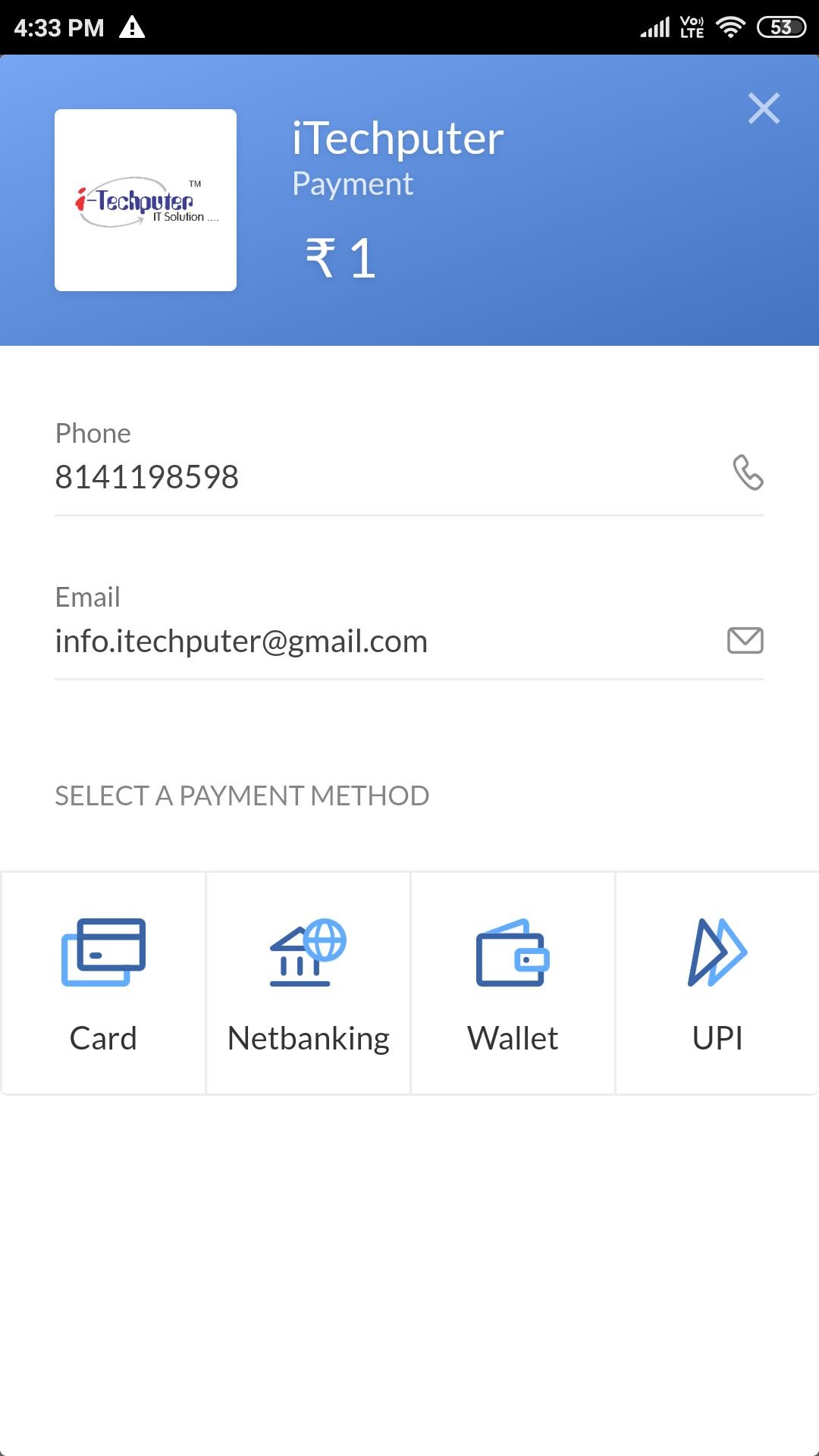The screenshot is taken from a smartphone at 4:33 PM, as indicated by the time display at the top of the screen. The notification bar shows full LTE signal strength, Wi-Fi connectivity, and a 53% battery life. A special notification with a triangle and exclamation point is visible.

The main content of the screen appears to be an online banking interface. The header reads "I-Tech Putter Payment," followed by an amount shown in a currency symbol resembling a capital 'R,' but with the left line removed and two horizontal lines at the top.

Below the text is the I-Tech Putter logo, though it is partially obscured by a watermark that makes the logo difficult to view. The watermark overlays a phone number, 814-119-8598, and an email address, info.itechputter@gmail.com.

The screen offers various payment methods including Card, Net Banking, Wallet, and UPI, giving the user multiple options to choose from for completing their payment.